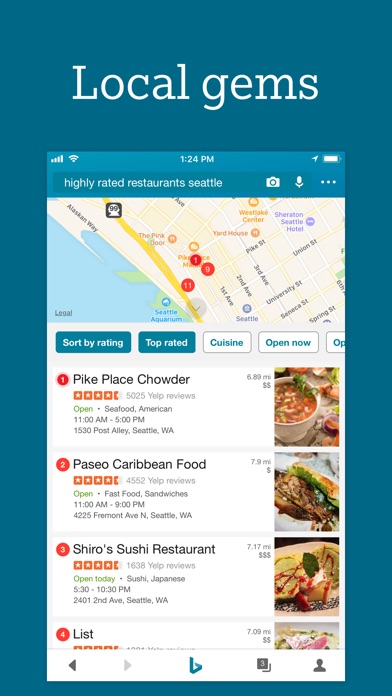Screenshot of a travel app interface displaying a search for "Highly Rated Restaurants Seattle." The background of the app features a dark navy blue color with the header text "Local Gems" in white. The central part of the screenshot shows a phone screen with the status bar indicating it is 1:24 p.m., a nearly full battery charge, and full Wi-Fi connectivity.

At the top of the phone screen, there's a search bar with the query "Highly Rated Restaurants Seattle." Below the search bar, the top three search results are displayed:

1. **Pike Place Chowder**
   - Rating: 4.5 out of 5 stars
   - Reviews: 5,220
   - Distance: 6.69 miles away

2. **Paycel Caribbean Food**
   - Rating: 4.5 out of 5 stars
   - Reviews: 4,552
   - Distance: 7.9 miles away

3. **Shira's Sushi Restaurant**
   - Rating: 4.5 out of 5 stars
   - Additional details suggest it is closer than the Caribbean food restaurant.